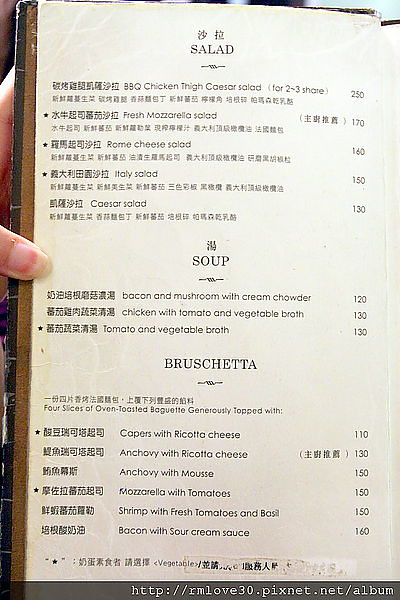A photo capturing a bilingual menu, featuring a range of delectable dishes organized into three sections: Salads, Soups, and Bruschetta. The menu is written in both Chinese and English. Under "Salads," the options include BBQ Chicken Thigh Caesar Salad, Fresh Mozzarella Salad, Rome Cheese Salad, Italy Salad, and Caesar Salad. The "Soup" section offers hearty choices such as Bacon and Mushroom with Cream Chowder, Chicken with Tomato and Vegetable Broth, and Tomato and Vegetable Broth. Lastly, the "Bruschetta" section presents several toppings, all served with four slices of oven-toasted baguette. The topping choices are Capers with Ricotta Cheese, Anchovy with Ricotta Cheese, Anchovy with Moose, Mozzarella with Tomatoes, Shrimp with Fresh Tomatoes and Basil, and Bacon with Sour Cream Sauce. The bottom of the menu includes a watermark: http://rmlove30.pixnet.net.